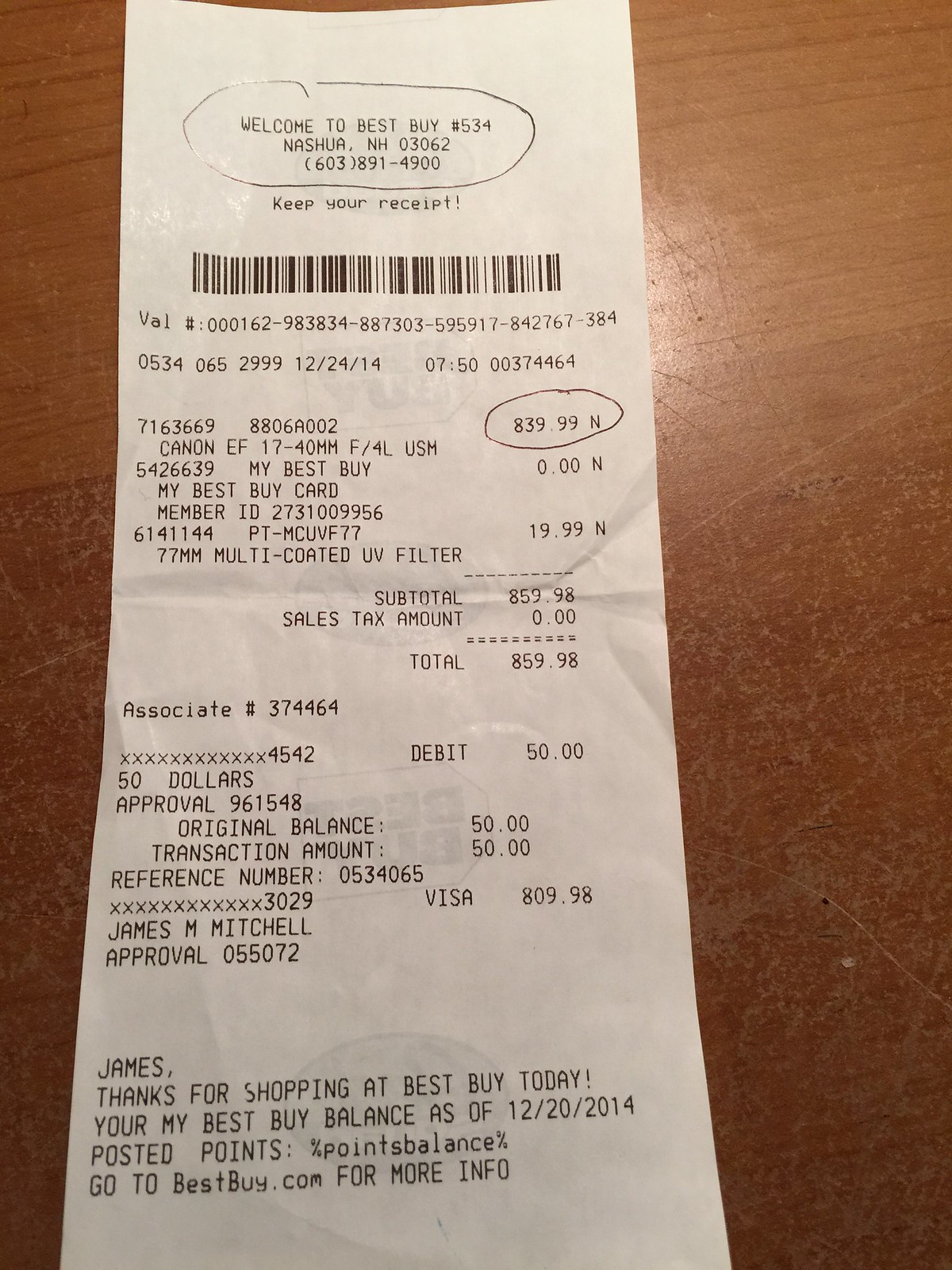The photograph showcases a receipt from a Best Buy store, neatly positioned on a light brown tabletop with distinctive distressed gray markings and scratches. Prominently featured at the top of the receipt, circled in ink, is the welcoming message: "Welcome to Best Buy, number 534, Nashaw, New NH, 03062603891-4900." Below, a circled item costs $839.99, indicating a purchase of a "Canon EF17-40mm f/4L USM," a high-quality camera lens. The receipt further notes a separate purchase of a multi-coated UV filter priced at $19.99. The total amount for both items is $859.98. Payment details reveal $50 was paid via debit card and the remaining balance of $809.98 was charged to a Visa card. Additionally, the receipt includes a $0 charge from the customer's Best Buy card, member ID 2731009956, and is associated with employee number 374464.